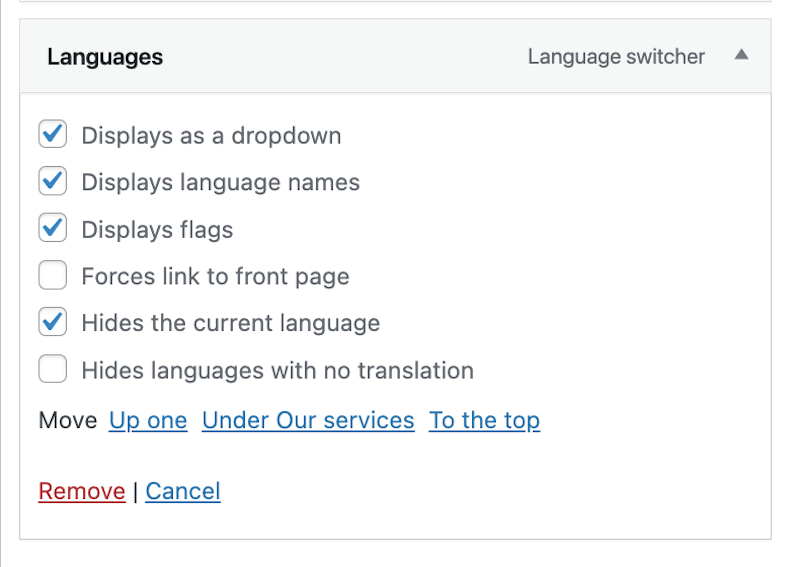**Caption:**

The screenshot captures a cropped segment of a menu focused on adjusting language preferences within an unspecified application. The image prominently displays a gray-bordered box, featuring a header bar at the top. The background of the header is gray, with "Languages" written in bold black text on the left and "Language Switcher" along with an up arrow icon on the right, indicating the presence of a clickable dropdown menu. 

The main portion of the box has a white background and includes several settings options equipped with checkboxes. The options displayed are:
- "Displays it as a drop-down" (checked on)
- "Displays language name" (checked on)
- "Displays flags" (checked on)
- "Forces link to prevent page" (unchecked)
- "Hides the current language" (checked on)
- "Hides language with no translation" (unchecked)

Below these checkboxes, there is a list of horizontal options for managing the order of languages or preferences:
- "Move" (currently selected)
- "Up one" (clickable)
- "Under our services" (clickable)
- "To the top" (clickable)

Finally, at the bottom of the box, there are two additional options, "Remove" and "Cancel", indicating actions the user can take regarding their language settings.